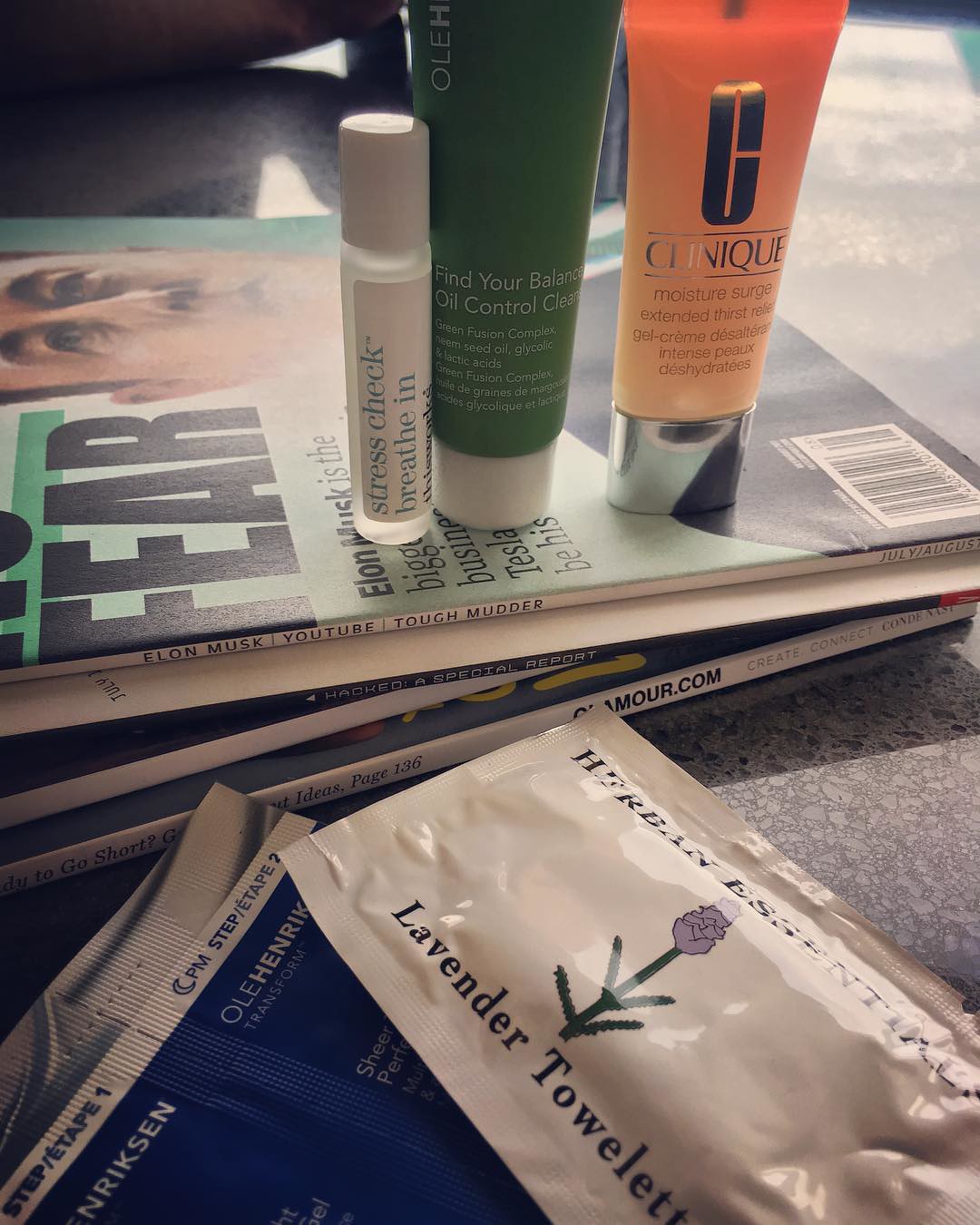On the table in the image sits a collection of magazines adorned with various skincare products. There are four skincare items in total: three tubes and one towel product. The three tubes rest on top of the magazines, while the towel product is placed directly on the table. 

Each of the tubes is distinctly labeled. The first tube reads, "breathe in." The second tube, positioned in the middle, is marked with, "find your balance, oil control, cleanser, Grain Fusion Complex, Nameseed Oil, Glycolic, Lactic Acid, Grain Fusion Complex," followed by a text in another language. The third tube, on the right, displays, "clinic, moisture surge, extended thirst relief, gel," with additional text in what appears to be French.

The scene is accented by a variety of colors, including green, black, white, orange, blue, and grey, adding to the visual interest of the composition.